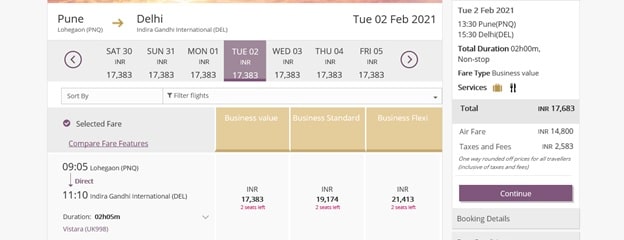Flight Information Screen for Pune to Delhi

The image displays a flight information screen detailing travel options from Pune (PUN) to Delhi (DEL). The title at the top reads "Pune to Delhi," with "Delhi" clearly highlighted, indicating an international destination.

Below the title, there are details listed for multiple travel dates:

- **Saturday, 30 INR**: 17,383
- **Sunday, 31 INR**: 17,383
- **Monday, 1 INR**: 17,383
- **Tuesday, February 2, 2021**: 17,383 (Highlighted in purple, suggesting it is the selected date)
- **Wednesday, 3 INR**: 17,383
- **Thursday, 4 INR**: 17,383
- **Friday, 5 INR**: 17,383

Each date has a circular icon next to it, with the purple circle signifying the selected date of Tuesday, February 2, 2021. On a gray background, there's a backward arrow in a circle, likely indicating a navigation option.

Below the dates, there's an option to "Sort by and filter flights," followed by "Select fare," which is highlighted with a purple circle that matches the selected date indicator.

Further down, there's a feature to compare fare options, with details including:

- **Time**: 9:05 PM
- **Flight Number**: (Possibly P & Q or D & Q)
- **Travel Type**: Direct
- **Arrival**: 11:10 PM at Indira Gandhi International (DEL)
- **Duration**: 2 hours and 5 minutes